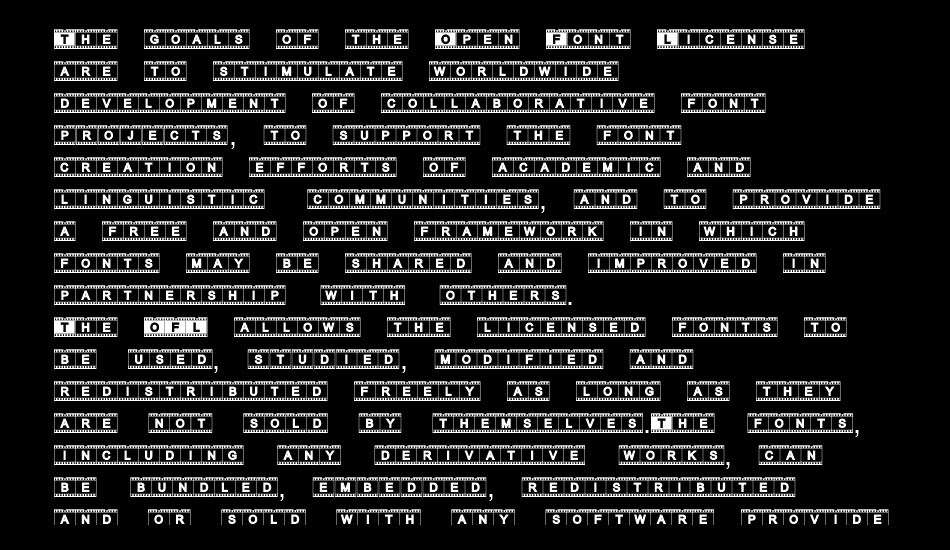The image features a black background with white, capitalized text. At the top and bottom of the text block, there are distinct border lines composed of closely spaced, small vertical lines. 

The text begins with the word "THE," where the letter 'T' has a white background contrasting with the rest of the black background. The caption then continues with "GOAL of the Open Font License," where the first letter of each of these words ("G," "O," "L") also has a white background.

Below this heading, there is a detailed explanation, stating: "The goals of the Open Font License are to stimulate worldwide development of collaborative font projects, support the font creation efforts of academic and linguistic communities, and provide a free and open framework in which fonts can be shared and improved in partnership with others."

The description concludes by highlighting: "The OFL allows the licensed fonts to be used, studied, modified, and redistributed freely, provided they are not sold by themselves. Fonts, including any derivative works, can be bundled."